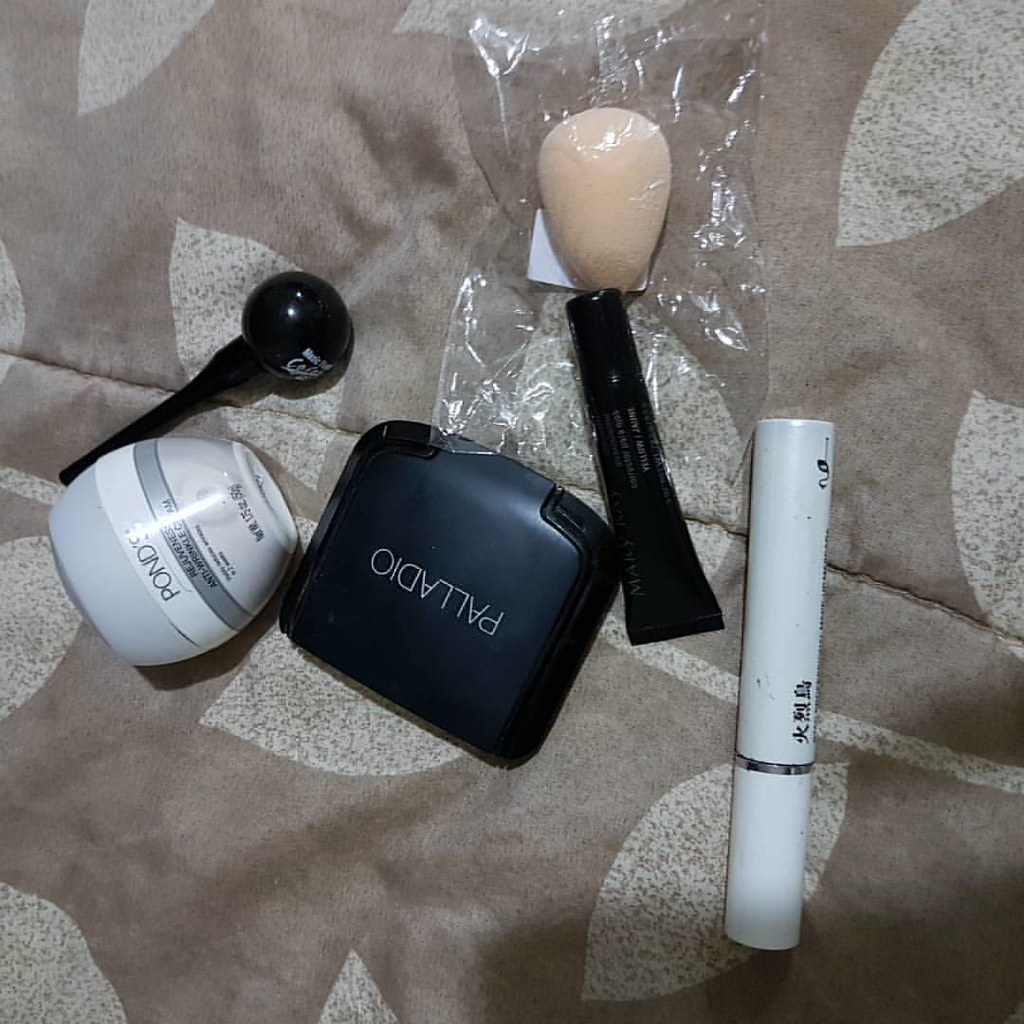The upside-down image features a collection of skincare items meticulously arranged on a brown blanket adorned with a pattern of white leaves. In the upper left corner, there is a sleek black bottle with a globe-shaped bottom and an elongated neck, devoid of any visible label. Below it, a round bottle of Ponds skincare product is prominently displayed, characterized by its gray cap, white body, and a distinctive gray band running vertically down the center. 

Adjacent to the Ponds bottle on the right is a compact, square black container that seemingly has an opening lid, with the brand name "PALLADIO" inscribed on it. Above this, a clear plastic bag contains a beige sponge at the top, accompanied by a black tube within. 

Positioned towards the bottom right, a white cylindrical product, likely an eye care item, stands out with its minimalist design. The cylinder features a white top and bottom, separated by a thin silver band, which likely represents the cap of the product.